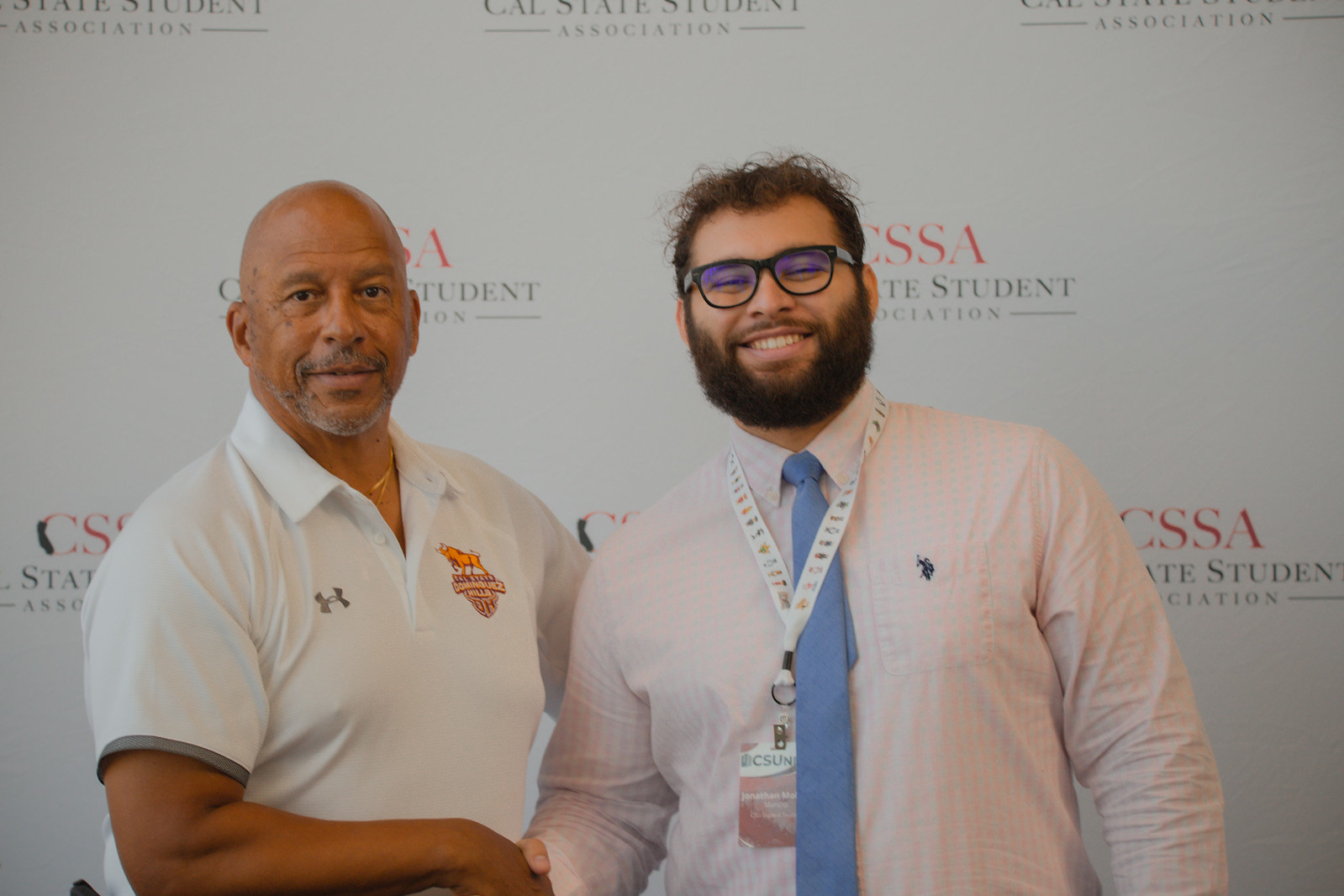In this detailed photograph, two men are posing in front of a backdrop covered with a repetitive logo. The logo features the letters "CSA" in red, with "Cal State Student Association" written underneath in black. Positioned against this backdrop, the two men are shaking hands and facing the camera, highlighting their friendly gesture. 

On the left, the man wears an open-collared white polo shirt paired with a silver and gold necklace. His attire is simple yet professional, complementing the formal setting. 

To his right stands another man, distinguished by his beard, mustache, and green and black-framed glasses. He sports a pink and white striped button-down shirt, accessorized with a white lanyard that holds a vertically oriented rectangular credential. His blue tie adds a touch of formality to his approachable look, while his slightly tousled hair adds to his charismatic appearance. This well-composed shot captures their camaraderie and the professional environment of the Cal State Student Association event.